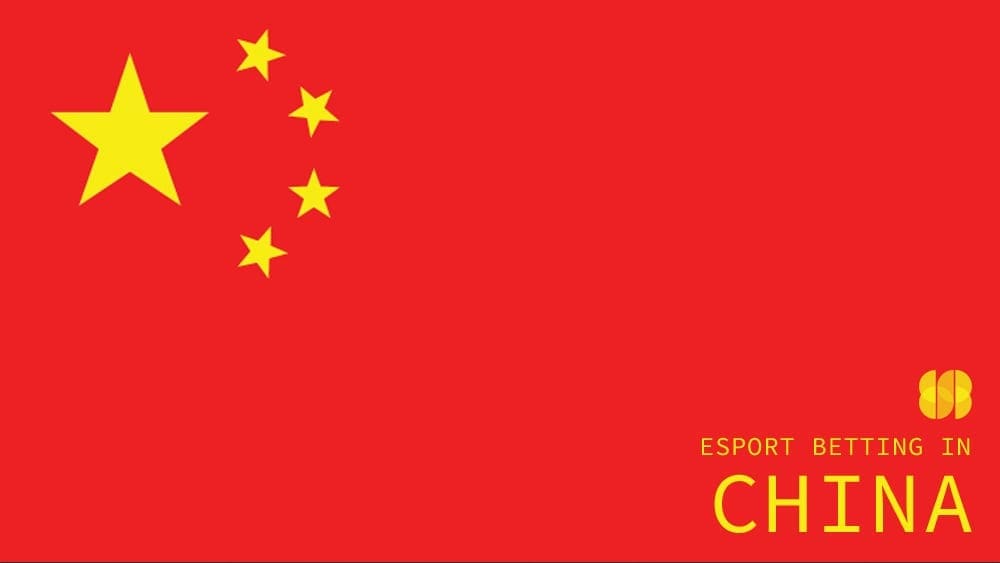The image depicts a horizontally oriented rectangular graphic with a prominent red background. In the top left corner, there is a large yellow five-pointed star, with four smaller yellow stars arranged in a semicircle around it, reminiscent of the flag of China. The bottom right corner features the text "eSport betting in China" in yellow, with the word "China" in larger block letters. Above this text is a company logo consisting of a design with three circles, one of which is halved, all rendered in yellow. The overall design is minimalistic and striking, dominated by its red and yellow color scheme.